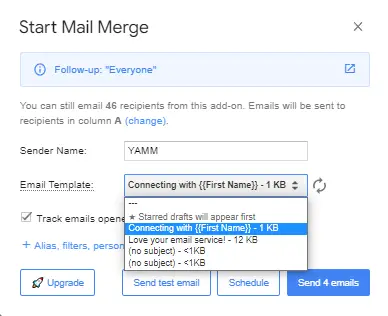Screenshot depicting a user interface on a light gray background. The interface features the following elements:

1. **Start Mail Merge with an "X" Icon**: Located at the top, used to close the mail merge function.
2. **Follow-Up Option**: Encased in quotation marks, likely a feature for following up with recipients.
3. **Visibility Icon ("Eye" in Circle)**: Indicates visibility options.
4. **Share Icon (Square with an Arrow Pointing Diagonally Upwards and to the Right)**: Suggests options to share the mail merge activity.
5. **Notification Text**: 
   - "You can still email 46 recipients from this add-on. Emails will be sent to recipients in column A."
   - "46" is bolded.
   - "A" is bolded.
   
6. **Change Option**: Displayed in blue text within parentheses, likely for modifying settings or selections.
7. **Sender Information**:
   - "Sender Name: YAMM" (all capital letters indicating the sender platform).
8. **Email Template Selection**: 
   - Dropdown list with templates titled "Connecting with [first name] - 1KB," "Love Your Email Service! - 12KB," and another unnamed template "<1KB."
   - The "Connecting with [first name] - 1KB" template is highlighted in blue.
   - Templates are shown with their respective sizes and an option to start drafts.
   
The entire interface indicates a detailed setup for managing and customizing mass email communications.